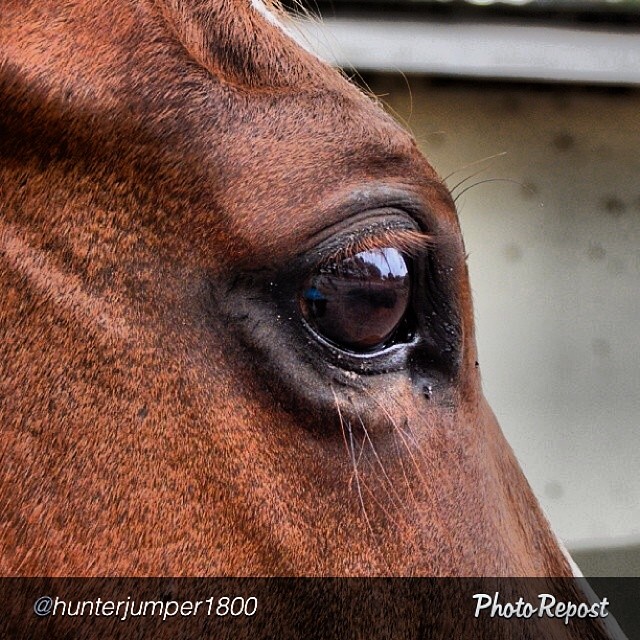This detailed, squared-format color photograph captures a close-up profile view of a horse's eye and surrounding features. The horse's reddish-brown hair and dark brown eye dominate the frame, with the focus being on the eye itself. You can see its long, brown eyelashes and a part of its forehead and snout. The image reveals a reflection in the horse's eye, suggesting it was taken outdoors, possibly during the daytime. The background is blurred and features a white-toned backdrop with an indistinct building to the right. A black strip overlays the bottom of the photo, containing white text that reads "at Hunter Jumper 1-800" on the left, and "photo repost" on the right. The photograph is marked by a realistic and detailed representational style.